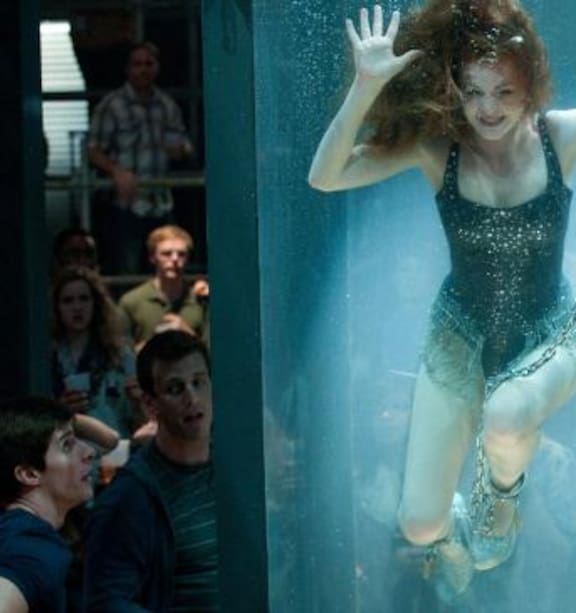The image depicts a dramatic, underwater scene of a woman performing what appears to be a Harry Houdini-style escape act. She is submerged in a transparent tank that is lit from below, creating a striking visual effect. The woman, who is Caucasian with long, brownish-red hair, is wearing a sparkly blue one-piece show outfit adorned with shoulder straps and lace, creating a skirt-like appearance that covers the top of her legs. Both of her hands are pressed against the glass, with one handcuffed and chained to her ankles, which are also shackled. Her knees are pulled up towards her body, and she appears to be intensely focused on her escape. Two onlookers are visible on the left side of the image, observing the captivating scene from outside the tank. The photo, taken in an indoor setting, features a color palette that includes off-white, black, gray, silver, emerald green, and hints of rust red, adding to the theatrical atmosphere of the picture.